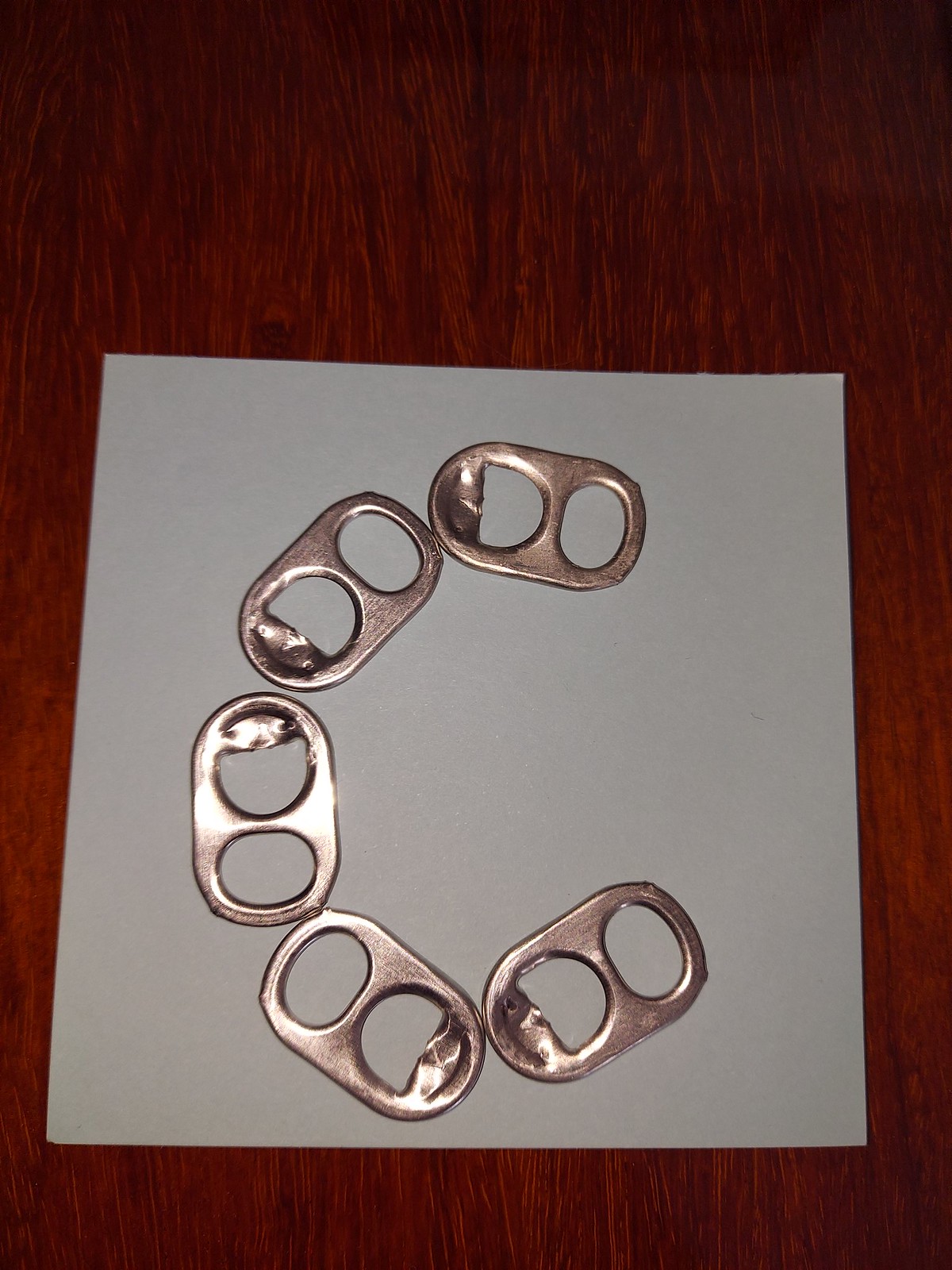This image captures a close-up view of five soda can pull tabs carefully arranged in a C-shape formation on a square piece of gray paper. The gray paper rests on a vibrant cherry-red wooden surface, whose texture is clearly visible in the photograph. The pull tabs appear freshly removed from cans and are positioned so that each one touches the next, forming a distinct crescent. Under the illumination of flash photography, the silver or subtly rosy-tinted tabs exhibit a shiny reflection, particularly from the tabs on the lower left. Although they seem to be simply placed rather than glued, the precise arrangement suggests a deliberate composition.